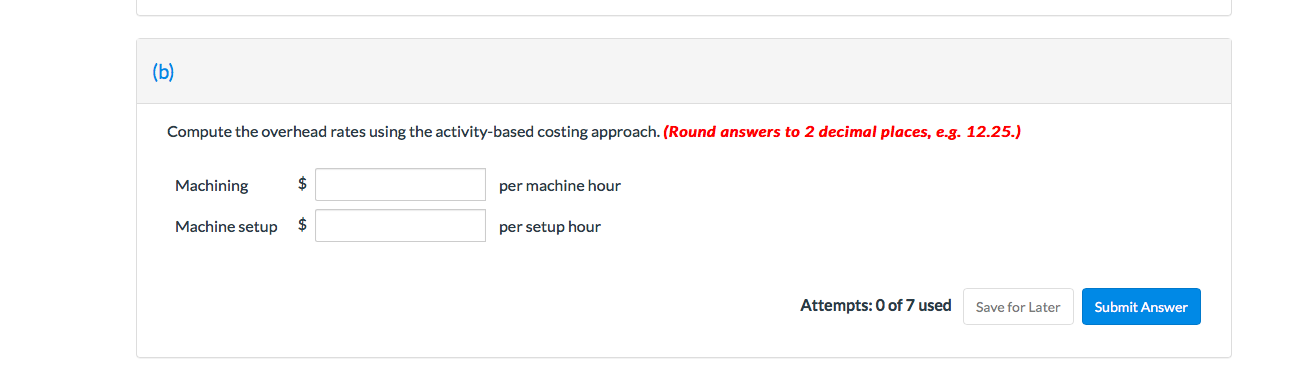The webpage displays a segmented layout, likely part of a larger website, as indicated by the letter "B" in blue parentheses positioned in the upper left corner, suggesting this is section B of a multi-part resource. The page header, highlighted by a shaded gray bar that extends across the width of the screen, reads "Section B." Beneath this, in bold black letters, is the directive: "Compute the overhead rates using the activity-based costing approach."

Additional instructions are provided in red text, emphasizing the need to round answers to two decimal places, with an example format of "12.25" indicated in parentheses. Below these instructions, two input bars are presented: one for "Machining," with a label for cost entry in dollars per machine hour, and another for "Machine Setup," also with a cost entry field designated in dollars per setup hour.

At the bottom of the webpage, a status message indicates "Attempts 0 of 7 used," accompanied by two interactive buttons: a white "Save for Later" box and a prominent blue "Submit Answer" box with white text, ready for user interaction. The page design is compact, focused, and aimed at guiding the user through the specific task of computing overhead rates.